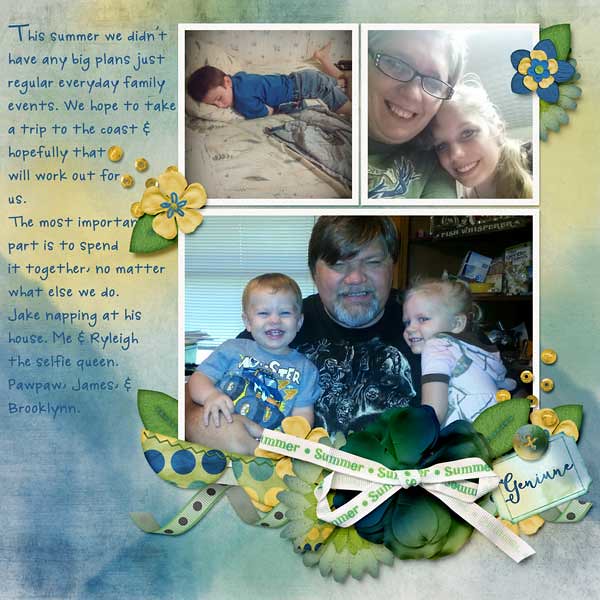This digital photo collage captures the heartwarming essence of a family's summer moments, emphasizing togetherness over grand plans. The layout features three photographs brimming with family love and decorative flair. 

At the top left, a young boy named Jake naps peacefully, dressed in a blue t-shirt and jean shorts as he lays face-down on his bed, one leg playfully raised. Adjacent to this, on the right, a touching photo showcases two blonde women—one smaller and skinnier, the other wearing glasses. They share a tender moment as the younger female, Riley, rests her head on the older woman's shoulder, their smiles radiating warmth and joy.

Beneath these, a broader image presents a man in his late 20s to early 30s, sporting a closely cropped beard and short haircut, holding two children—possibly twins. The boy in his right arm beams with a big smile, wearing a blue t-shirt, while the girl in his left arm, clad in a white outfit, exudes a charming, gentle smile. This family scene exudes genuine affection and delight.

Accompanying these cherished images are ornate 3D floral designs, adding a whimsical touch. Below the family photo, a detailed cloth representation of flowers features a green flower with a white ribbon inscribed with "summer" wrapped around it. A ticket stub-like design in the lower right corner reads "genuine," enhancing the collage's nostalgic feel.

To the left of the images, a heartfelt message in a handwritten-style font reads: "This summer we didn't have any big plans, just regular everyday family events. We hoped to take a trip to the coast, and hopefully that will work out for us. The most important part is to spend it together, no matter what else we do." The caption lovingly identifies the family members: "Jake napping at his house, me and Riley, the selfie queen; Pawpaw, James, and Brooklyn."

This composition, with its pastel hues of greens and yellows, intricate floral embellishments, and personal touch, captures the essence of a scrapbook page, celebrating the joy and simplicity of family life.